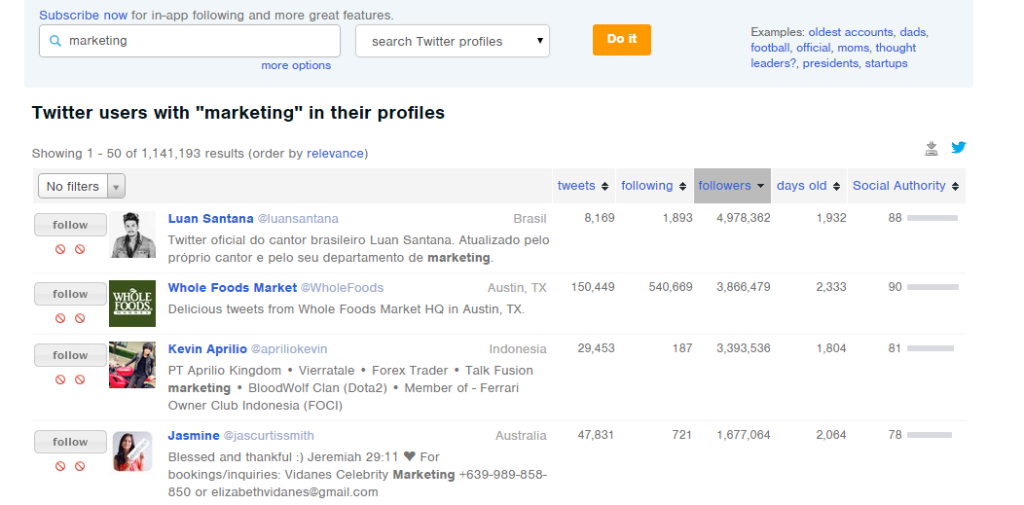This is a detailed screenshot from a website that aggregates information, specifically focused on the app Twitter. At the top of the page, there's a very faint blue banner. On this banner, "Subscribe now for in-app following and more great features," is prominently written in blue. Below the banner, there's a search box with the term "marketing" typed in black. To the right of the search box is a drop-down menu set to "search with their profiles." Next to this drop-down, there's a distinct orange button with "Do it" written in white, which presumably initiates the search function.

On the far right of the banner, various categories such as "examples," "oldest accounts," "dads," "football," "official moms," "thoughts," "leaders," "presidents," and "start-ups" are listed. Beneath this banner, the page displays the heading: "Twitter users with 'marketing' in their profiles." It notes that there are 1.141 million results, showing entries 1 to 50, sorted by relevance.

The results start with accounts ranging from Luan Santana to Whole Foods Market, Kevin Aprelijo, and Jasmine. These accounts are geographically varied, from Brazil, Austin, Texas, Indonesia, to Australia. The number of tweets per account is also detailed: Whole Foods Market leads with 150,449 tweets, followed by Jasmine with 47,831, Kevin Aprelijo with 29,453, and Luan Santana with 8,169 tweets. Additional information such as the number of followers, days the account has been operational, and social authority scores are provided for each account.